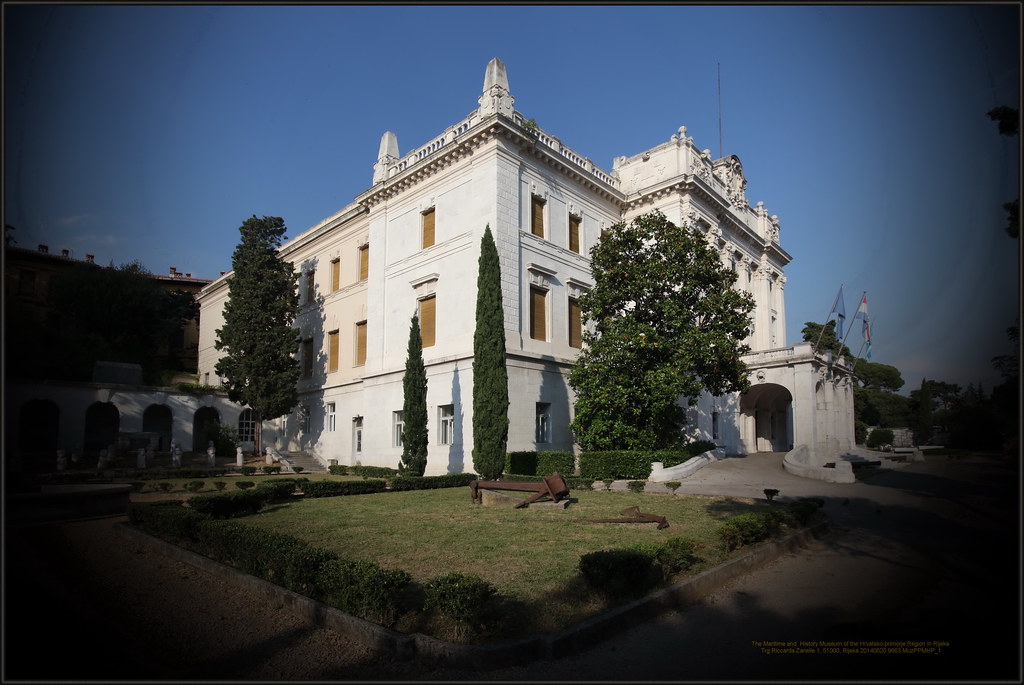This photograph showcases a stately and professional three-story building, likely with political or diplomatic significance, possibly an embassy. Viewed from a corner angle, the building stands out with its white facade and amber-brown windows, which are either adorned with gold curtains or boarded up. The entrance is marked by a covered archway supported by pillars, leading up to a pathway with a gentle ramp. Three flags are prominently displayed above a porch or patio area, reinforcing its formal nature. The grounds around the building are meticulously maintained, featuring a well-kept garden with shrubs and groomed trees. Additional embellishments such as elegant engravings and elaborate roof detailing add to the building's historic and dignified appearance.